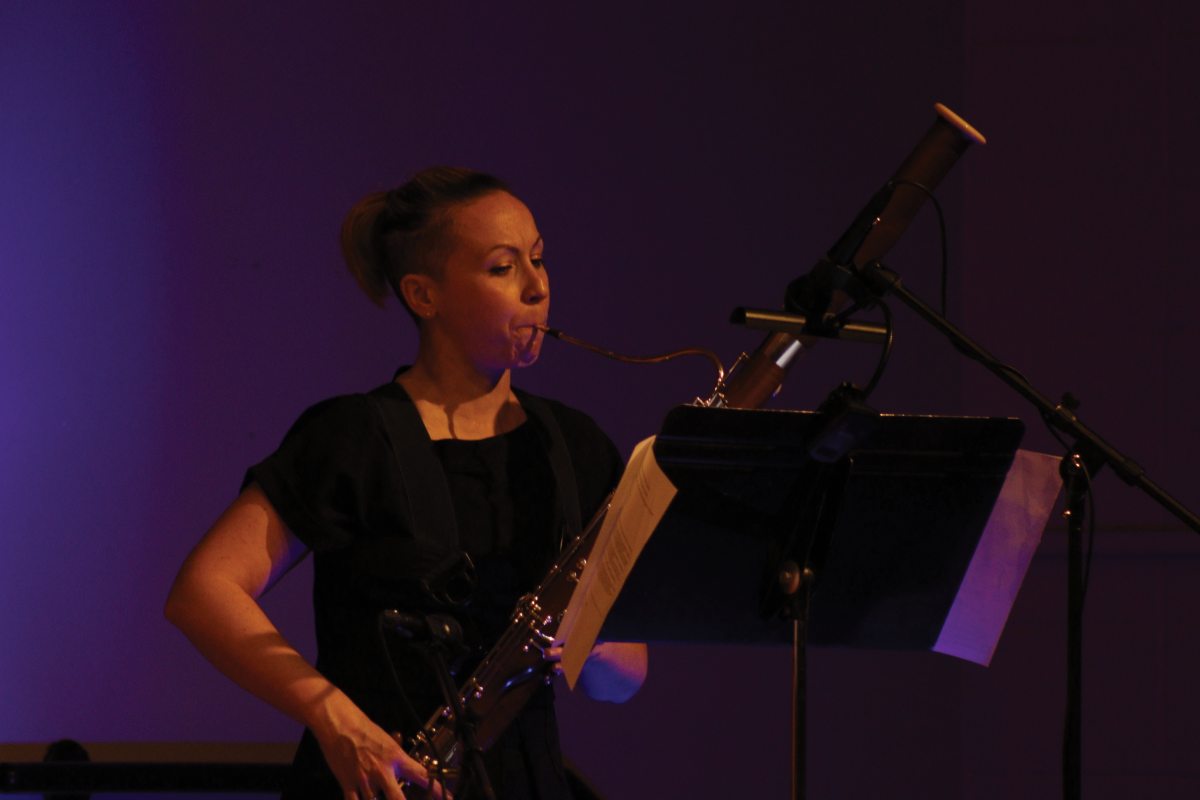The full-color, horizontally rectangular photograph, taken indoors with artificial lighting, features a young Caucasian woman performing on stage. The background consists of various shades of purple, illuminated by the stage lights, creating a visually compelling scene. The performer, dressed in a dark top with short sleeves, stands confidently with one side of her head shaved and her short blonde hair pulled back into a ponytail. 

She is playing a bassoon, which is a tall, black woodwind instrument with a slender, long tube extending from its side into the mouthpiece, and her hands are skillfully placed on the instrument's valves. The bassoon slopes at a 45-degree angle as she plays, with her lips tucked under to reach the reed. To her right, a music stand holds her sheet music, and a light affixed to it aids her performance while a microphone mounted on a black stand captures the sound. Her body faces forward, but her head turns toward the music stand, fully engaged in the act of reading the music and playing simultaneously. The stage setup includes subtle details such as a possible table on the left side of the image, contributing to the overall ambiance of the scene.